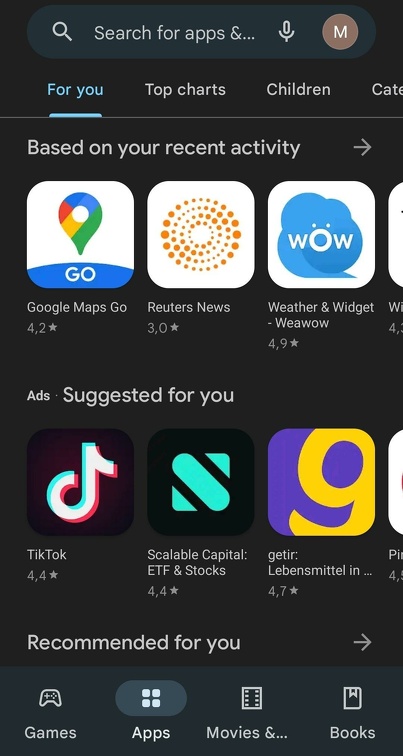The cropped image showcases a portion of a digital interface, possibly a smartphone or tablet screen. At the top, there is a brown-circled icon featuring a username that starts with a capital 'M'. Beneath this, a search bar labeled "Search for apps" is visible, though its contents remain unspecified. 

Highlighted tabs including "4U," "Top Charts," and "Children" suggest a personalized and categorized browsing experience, but other potential categories are cut off from view. The "4U" tab is emphasized, indicating it's the current view.

Under the "Based on your recent activity" label, several suggested applications appear: Google Maps Go, Reuters News, and an app for weather and widgets, among others. A section marked "Suggested for you" presents a series of advertisements, showing apps such as TikTok, Scalable Capital (ETF and stocks), and GETIR (partially displayed as "Liebensmittel"). 

Finally, a "Recommended for you" section points off to the right side of the screen, but the actual recommendations are not visible in the cropped image.